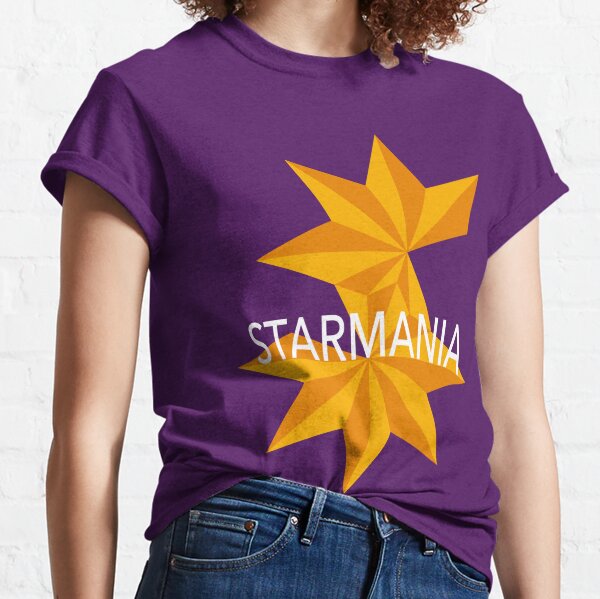The image depicts a young woman modeling a short-sleeved purple t-shirt that reads "Star Mania" adorned with two stars and some orange-tan polygon figures. The woman is seen from the neck down, showcasing her attire. She has curly red hair, which spills out of the frame's top edges. The t-shirt appears to be tucked into her blue jeans. The background is a white brick wall, giving a neutral setting focused entirely on the t-shirt. The woman is facing towards the right side of the image, with more of her hair visible on that side, suggesting she might be glancing towards the center of the image. The emphasis of the picture is entirely on her outfit, particularly the "Star Mania" t-shirt, with no other accessories or elements in view.